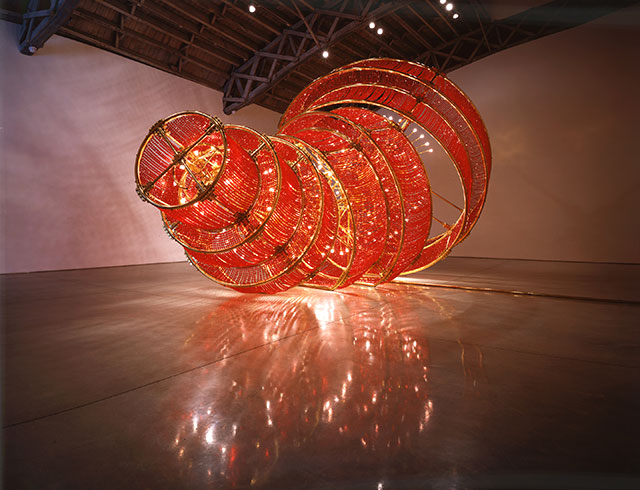This is a wide rectangular photograph of a large, intricate 3D art installation situated indoors. The image captures a striking, chandelier-like structure that resembles a cornucopia, laid on its side on a reflective gray floor consisting of large rectangular panels. The art piece, comprised of a vibrant cascade of crimson and orange beadwork suspended between gold hoops, forms a seven-layered tier that curves gracefully. The gold rims outline each circle and cross over one another, creating an elaborate, intertwined design. Small white light bulbs spiral throughout the structure, adding a mesmerizing glow. The ceiling is partially visible, showcasing wooden rafters and beams intersecting above, with open scaffolding and artistic low lighting. The bright white walls surrounding the installation cast subtle shadows, enhancing the dramatic effect of the reflection of the elaborate chandelier on the polished floor below. The overall scene is richly detailed, highlighting the meticulous metalwork and the captivating beauty of this art exhibit.